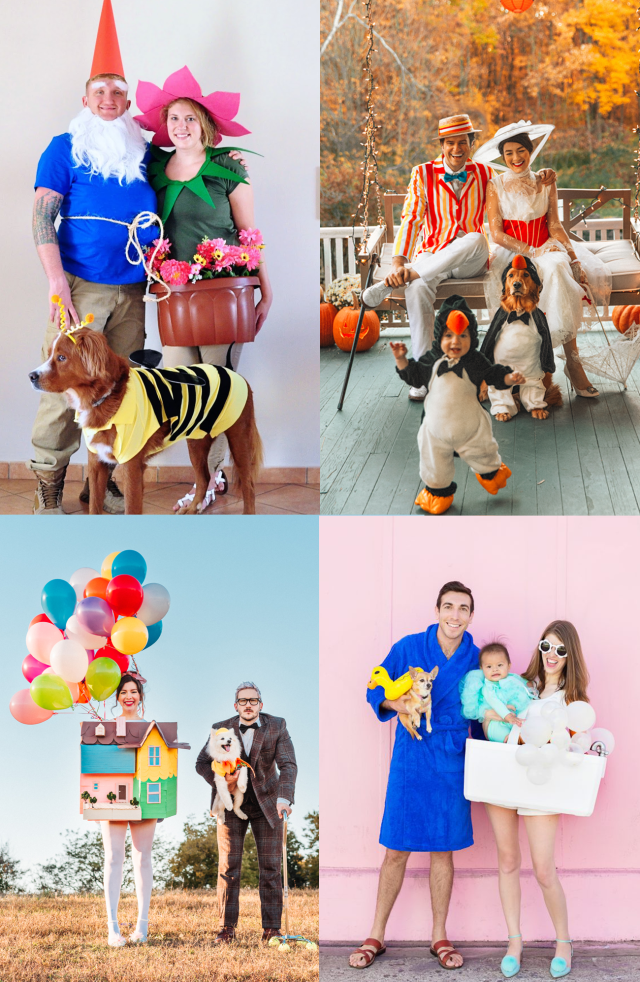This collection features four comedic, family-themed photographs of young couples in elaborate, themed costumes. Each photograph uniquely combines humor and whimsy, with both pets and children playing integral roles in the scenes:

1. In the upper-left photo, a man dressed as a gnome in a blue shirt, red hat, white beard, and bushy eyebrows stands beside a woman who is whimsically dressed as a flower emerging from a pot. She has a flowerpot around her waist, green leaf collar, and a flower bloom on her head. Their playful brown dog, dressed as a bumblebee, completes the ensemble.

2. Next to that, on the top-right, a couple poses with their toddler and dog against a backdrop of autumn foliage, reminiscent of characters from Mary Poppins. The man channels the Dick Van Dyke character with an orange and yellow striped suit jacket and matching hat, while the woman, in a large white hat and white dress with an orange belt, echoes the iconic Julie Andrews role. Both the toddler and the dog are charmingly dressed as penguins.

3. On the bottom-left, a humorous bubble bath scene features a man in a blue bathrobe holding a Chihuahua alongside a woman embodying a bathtub, complete with balloons as bubbles and a white basket-like bathtub around her. Between them, a baby is dressed adorably as a bath sponge with frilly material, set against a pink background.

4. The bottom-right photo brings the characters from the movie "Up" to life, with a woman dressed as a house, complete with balloons, standing beside a man portraying the old man from the movie, complete with a bowtie and glasses. They are accompanied by their dog, enhancing the whimsical outdoor setting.

Each photograph combines creativity, eccentric costumes, and a lighthearted family atmosphere to create memorable and strikingly vivid images.